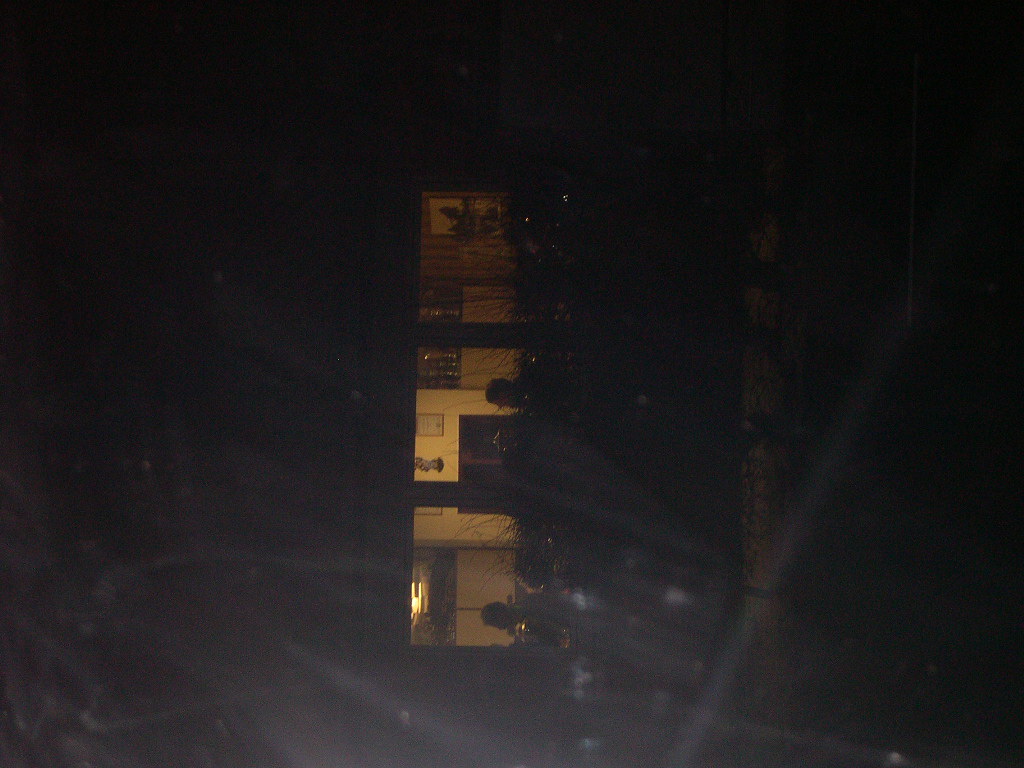A nighttime photograph capturing a scene through a dirty window. The exterior of the image is enveloped in darkness, punctuated by visible streaks and spots on the glass that suggest grime. Slightly to the right within the frame, a straight brown pole—a telephone pole—can be discerned, providing a subtle vertical element against the black backdrop. The photographer's gaze appears to be directed through the glass towards an interior space with three vertically aligned windows. Each window offers a glimpse into a different scene:

- In the bottom window, a head is visible in the lower right corner, with a white panel behind it, possibly indicating a door. There is also a darker area nearby.
- The middle window reveals what might be a flat-screen TV, accompanied by a head to the right of it and a picture hanging on the wall, contributing to a more discernible yet still enigmatic interior.
- The top window is more ambiguous, its contents lost to the shadows of the night.

The scenes inside these windows are bathed in a pale, yellowish light, casting a muted glow that contrasts against the surrounding darkness.